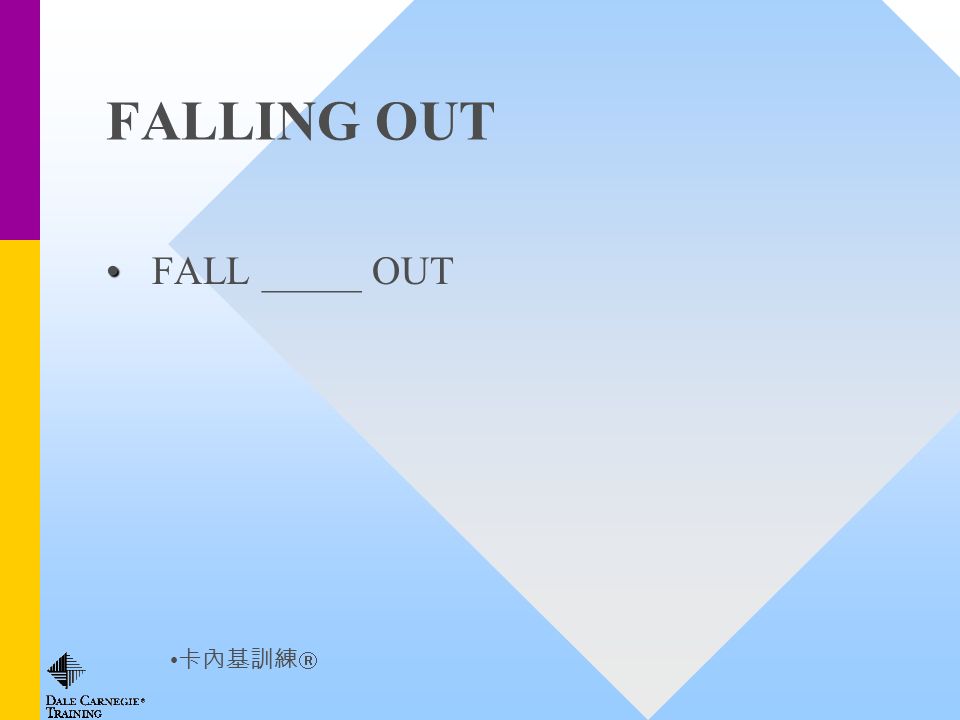The image is a presentation with a detailed layout. The background transitions from white at the top to blue at the bottom. On the left side, there is a vertical bar: the top third is purple, while the bottom two-thirds are dark yellow or gold. In the middle-right section of the image, there is a diamond shape with the top part cut off, featuring a light blue upper section that transitions into white at the bottom.

In the top left corner, there is a title in black capital letters that reads "FALLING OUT." Directly below it, a bullet point in a smaller font states "FALL _ OUT." Towards the bottom left corner, Chinese characters are visible, followed by the text "DALE CARNEGIE TRAINING." This text signifies the company logo. The elements are visually aligned and upright, creating a structured and cohesive presentation.